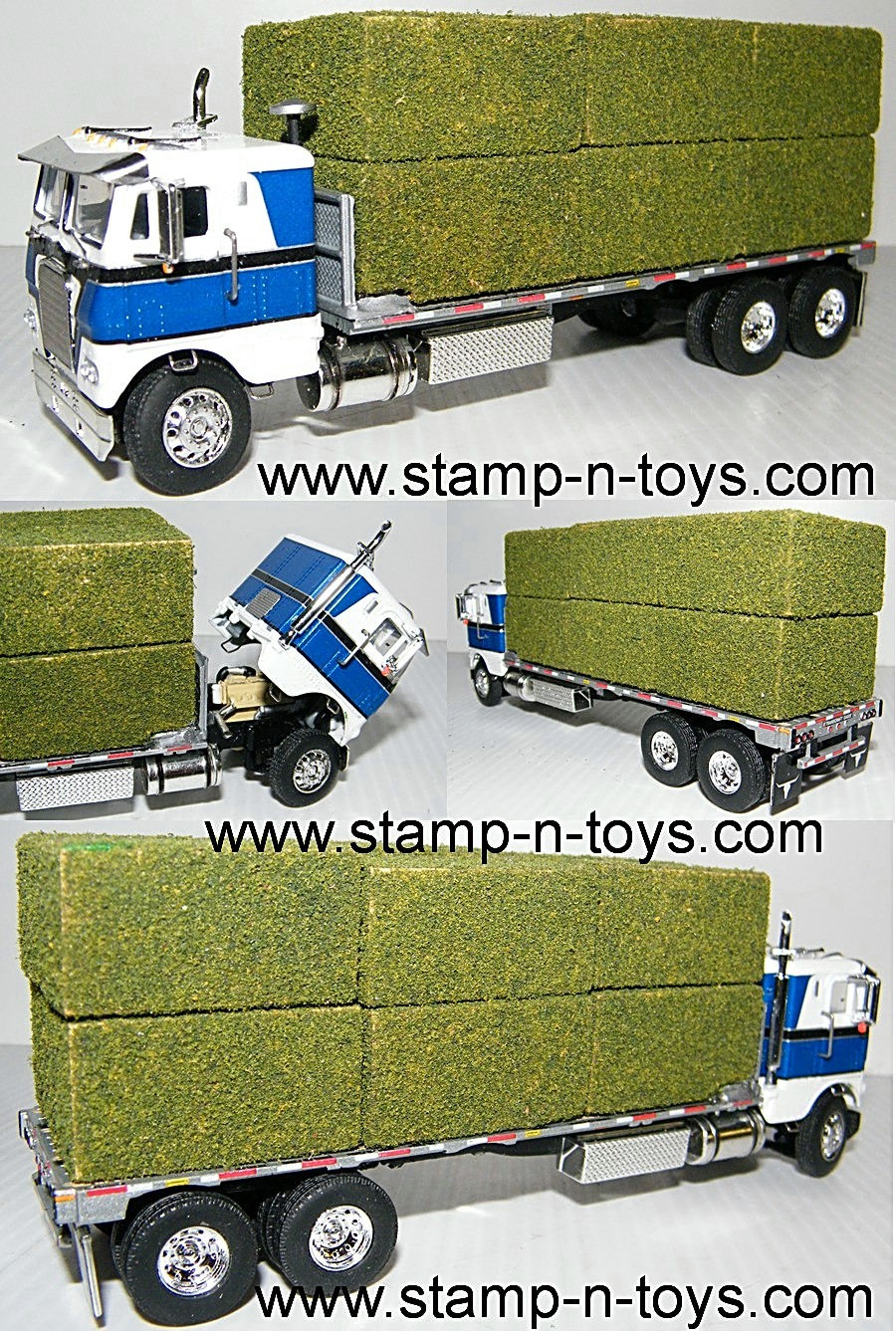This product image showcases four detailed photographs of a toy semi-truck, divided into three horizontal sections. In the upper third, the truck faces left, displaying its white cabin with a blue stripe and a total of six visible wheels, three on each side. Rectangular bales, resembling green and yellow hay, are stacked on its flatbed. The middle section features two images: one demonstrating the cabin's ability to tilt forward, exposing the engine, and the other capturing the truck from a rear perspective. The bottom third presents a right-side profile of the truck. Each section includes the website "www.stamp-n-toys.com" in black font.